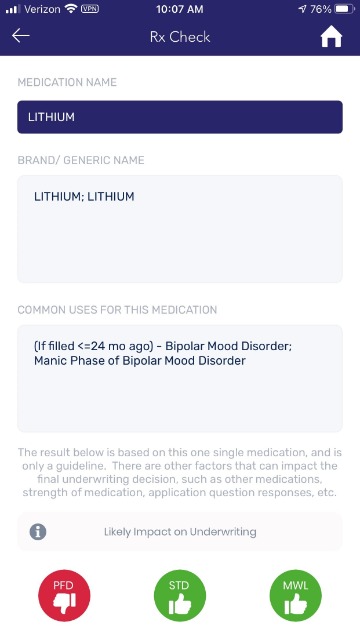The top of the image features a long bar in a purplish-blue hue with the word "Verizon" on the left. At the center of this bar, the current time is displayed as 10:07 AM, and to the right, the battery life is indicated at 76%. Directly below the time, the text "RX check" is present, with a capital 'R' and lowercase 'x'. Adjacent to this text on the right side is the symbol of a white house.

Beneath this section is a white area with very light gray text that reads "Medication Name." Below this, within a purple box featuring white capital letters, is the word "LITHIUM." Further down, the text "Brand/Generic Name" appears, followed by "Lithium; Lithium" in black text. Additionally, in gray text under this, there's information on the common uses for this medication, specifically noting "Bipolar Mood Disorder" and "Manic Phase of Bipolar Mood Disorder," with a reference to being filled 24 months prior.

Towards the bottom of the image, there are three circles with symbols and letters inside them: a red circle featuring a thumbs-down icon with the letters "PFD" in uppercase, a green circle to the right with a thumbs-up icon and the letters "STD," and another green circle to the right of that with the letters "ML," "MWL," and a thumbs-up icon.